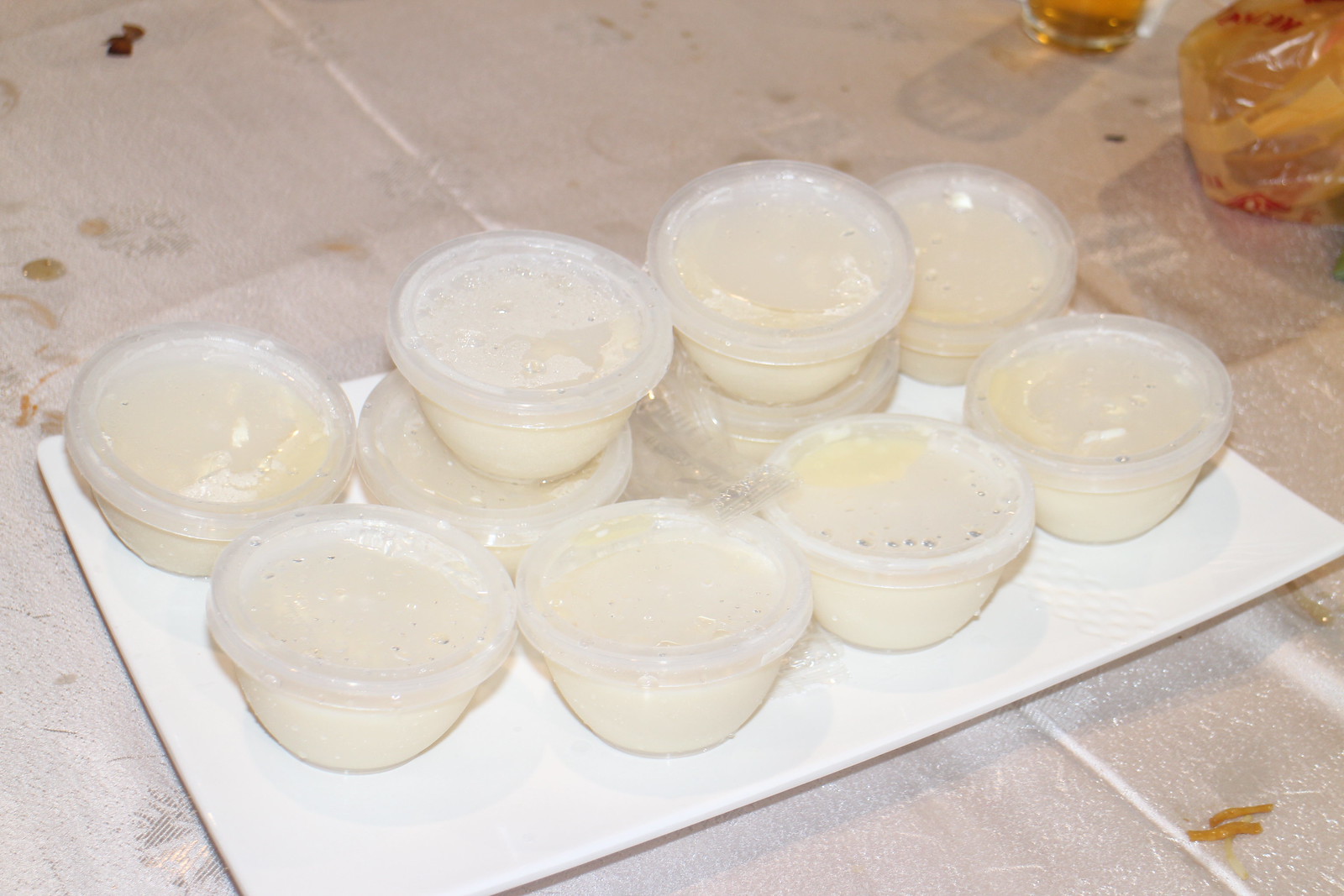This indoor photo features a white rectangular porcelain serving tray set upon a white tablecloth. The tray holds precisely ten small plastic dipping cups, each filled with a white sauce and secured with lids, showing signs of condensation. In the background, scattered on a tiled surface that appears somewhat dirty and stained, there are pieces of food and a drink containing a brown liquid, possibly beer or tea. The overall setting suggests a casual dining or food preparation area with additional food items or drinks visible in the surrounding space.